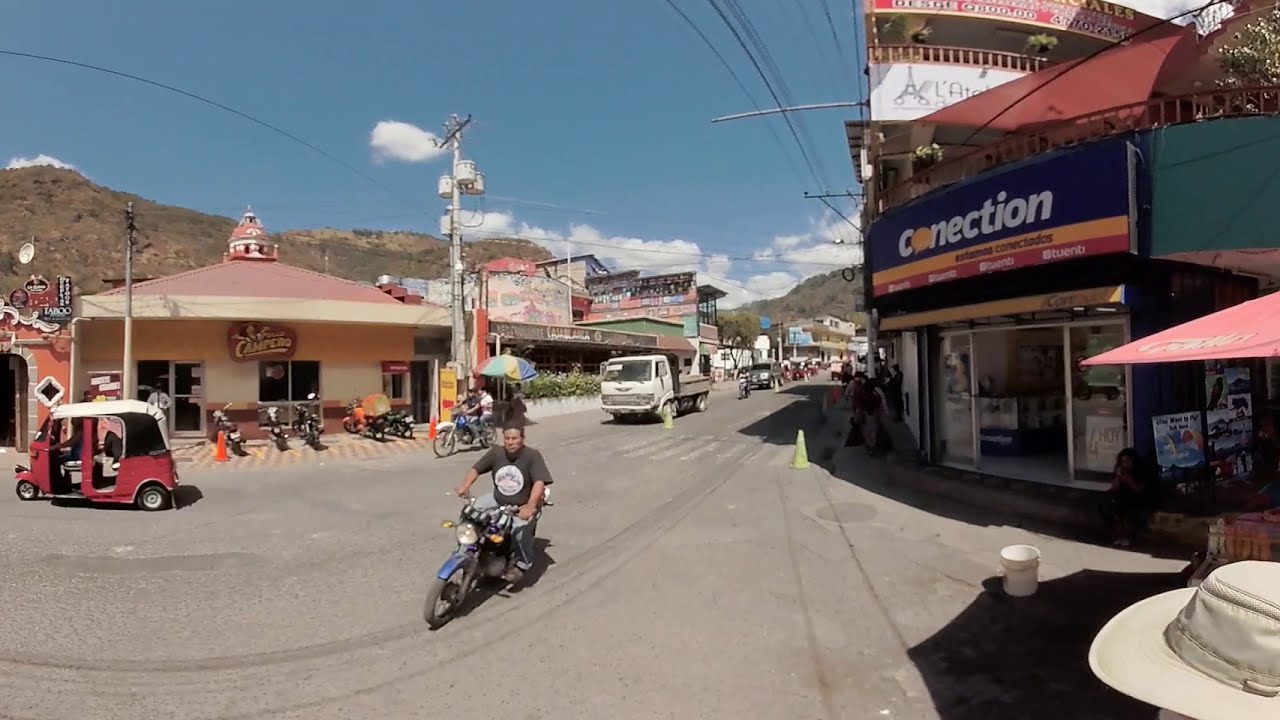The image captures a lively street scene in what appears to be a town in Mexico or South America, set outdoors in the middle of the day. The road, paved with gray asphalt, stretches into the distance, populated by several vehicles, including a prominent red taxi and a white truck, with numerous other cars trailing behind. Central to the picture is a man on a motorbike wearing a gray t-shirt with a white symbol.

To the right of the image, several storefronts and open-air eateries line the street. Notably, one store with an open door has a sign that reads "Connection" with "Conactitos" written beneath it. Next to this store, a light-colored hat is visible at the bottom right corner, though the person wearing it is not in view. An umbrella shades part of the right side, adding to the bustling atmosphere.

On the left side, you can see a hedge-bordered open-air restaurant and more shops, including one named "Camp Cito." Motorbikes are parked in front, contributing to the scene's dynamic nature. The far background reveals small, barren hills with stubby brown grass and a substantial portion of the blue sky filled with low-hanging clouds. Various colors dominate the image, including hues of blue, white, gray, red, orange, pink, black, and green, capturing the vibrant essence of this town.